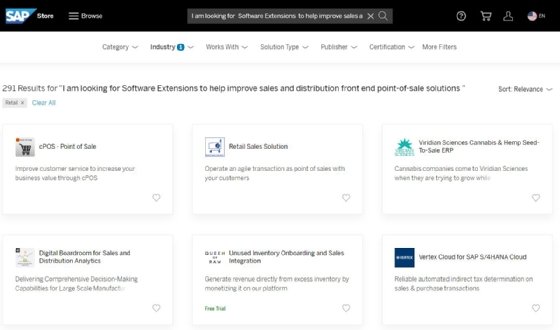This screenshot depicts the SAP Store interface, albeit slightly blurry, making the text somewhat challenging to read. At the very top, the header clearly displays "SAP Store," followed by navigation links "Browse" and a search bar, wherein the user has entered the query: "I am looking for software extensions to help improve sales..." The search query appears to be truncated.

Also in the header are several icons: a question mark for help, a shopping cart, a user profile icon, and a circular American flag labeled "EN" indicating the language selection is English. Below the header, on a white background, there are categorical filters that enable users to refine their search based on parameters such as "Category," "Industry," "Works With," "Solution Type," "Publisher," "Certification," and "More Filters."

The main content area reveals that the search query has yielded 291 results for software extensions aimed at enhancing sales and distribution front-end point-of-sale solutions. The results are sorted by relevance, as indicated. 

Beneath this summary, there are six highlighted rectangular sections, each representing a different software solution, complete with links and brief descriptions:
1. "CPOS Point-of-Sale"
2. "Sales Solution"
3. "Vinden Sciences"
4. "Cannabis and Hemp Seed Solutions"
5. "Digital Sales" (incomplete description)
6. "Unused Inventory"
7. "Vertex Cloud for SAP" 

Each of these solutions appears to cater to specific niches within sales and distribution enhancement.